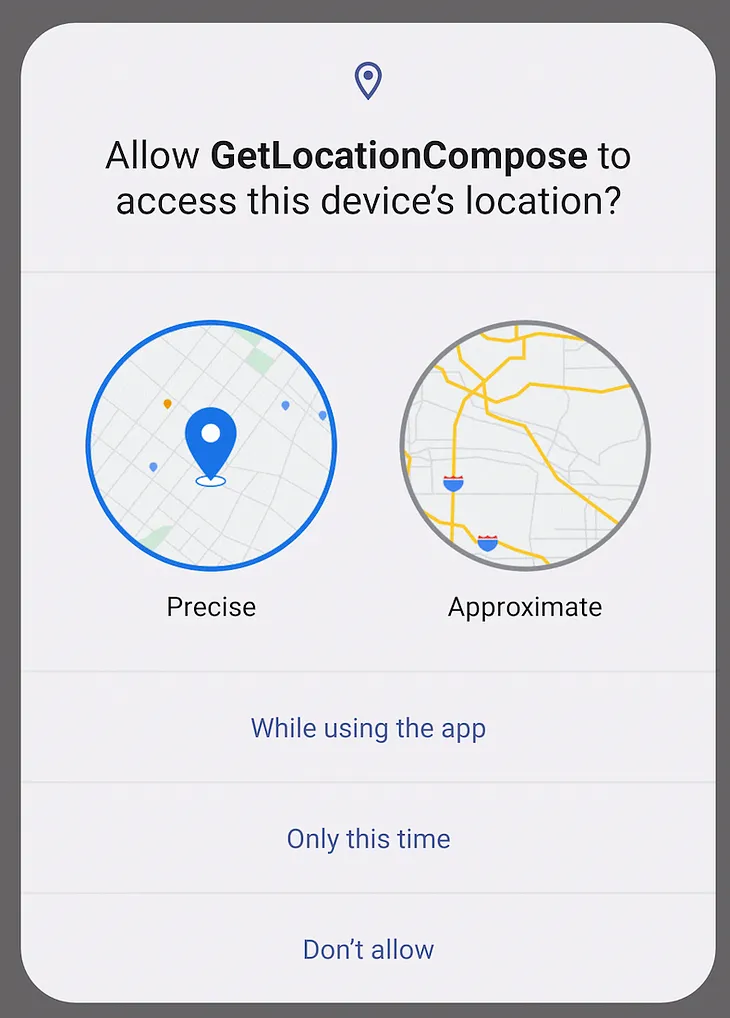This image appears to be a screenshot from a tablet interface displaying a permissions request for location access. The background of the interface is a dark gray, framed with four visible corners, and inside this frame, there is an inset rectangle with slightly rounded corners.

At the top-center of the rectangle is a blue pinpoint icon, resembling an upside-down teardrop with a circle, which typically represents a location marker. Below this icon, the text "Allow GetLocationCompose to access this device's location" is displayed. The application name "GetLocationCompose" is highlighted in a bolder black font, while the remaining text is presented in standard bold.

Underneath this prompt are two selectable options, each enclosed in circular icons:

1. The first option, highlighted with a blue ring, displays another blue pinpoint icon with a white center, situated on what looks like a simple map background. Below it, the word "Precise" is written, indicating that this option would allow precise location tracking.
2. The second option features a black circle containing a pattern of intersecting yellow lines, representative of a broader, less specific location. In the background of this circle, there are light gray lines and two highway sign symbols. Below this icon, the word "Approximate" is written, suggesting this choice would permit only approximate location data to be shared.

At the bottom of the screen, there are three different selectable options arranged in a list, each separated by light gray divider lines:

1. "While using the app" - indicated by a light gray line.
2. "Only this time" - following another gray line.
3. "Don't allow" - the last option, separated by an additional gray line.

This detailed layout prompts the user to make a choice regarding location permissions for the application in question, offering varying levels of location accuracy and frequency of access.